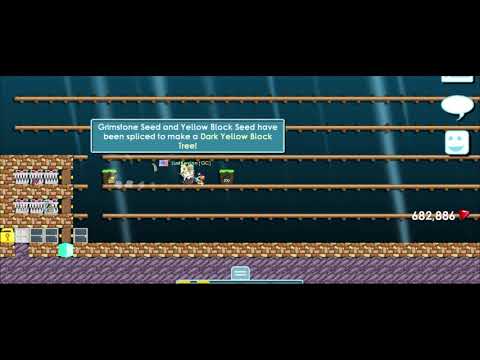A video game screenshot captures a vintage 2D side-scrolling game reminiscent of classic titles like Mario or Donkey Kong. The scene features a layered environment with five horizontal brown platforms or wooden planks extending across the screen. The top two planks span the entire width of the image, while the bottom three stretch from the right to connect with a brick building on the left. The background is a dark tealish-blue with white lines, giving it a nostalgic 8-bit appearance. Below the platforms, there's a purple base layer or street, and on the left side, a stone or brick building.

In the center of the image, a green text box reads, "Grimestone Seed and Yellow Lilac Seed have been spliced to make a dark yellow block tree." To the right, a score of 682,886 is displayed next to a red dot. The image also includes various characters located on the middle platforms, appearing to interact with each other. Additionally, the screen features letterboxes at the top and bottom, similar to a movie format, and a chat bubble with square icons on the right-hand side, next to the score. The prevalent colors in this scene are brown, purple, blue, yellow, green, red, white, and gray, contributing to the game's retro aesthetic.